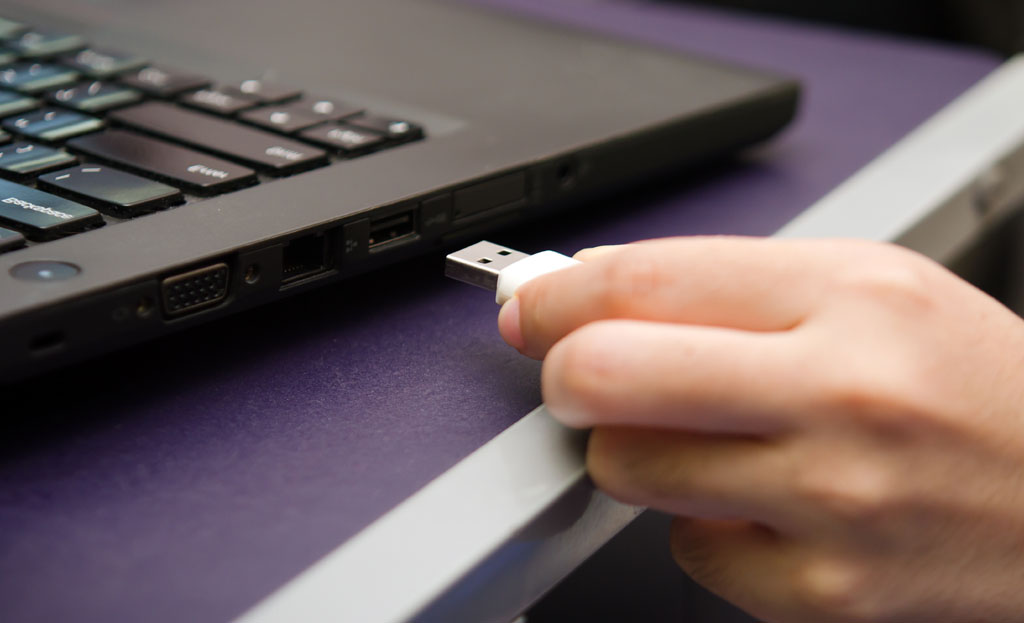This image captures a detailed close-up of a hand poised to insert a white USB drive into a black laptop. The upper left corner of the shot reveals the very edge of the laptop and its keyboard. The computer, which appears to be a PC, sits on a purple table with a distinct stainless steel edge near the hand. In the image's lower right corner, the person's hand can be seen holding the USB drive just an inch or two away from the USB port. The background behind the hand is predominantly black and extends to the upper right corner of the image. The laptop's placement is slightly angled rather than perfectly aligned with the table edge, and the hand, possibly a woman's due to its small size, bears no rings or fingernail polish, making it difficult to definitively identify the gender. The laptop itself features multiple ports, indicative of being a non-Mac device.